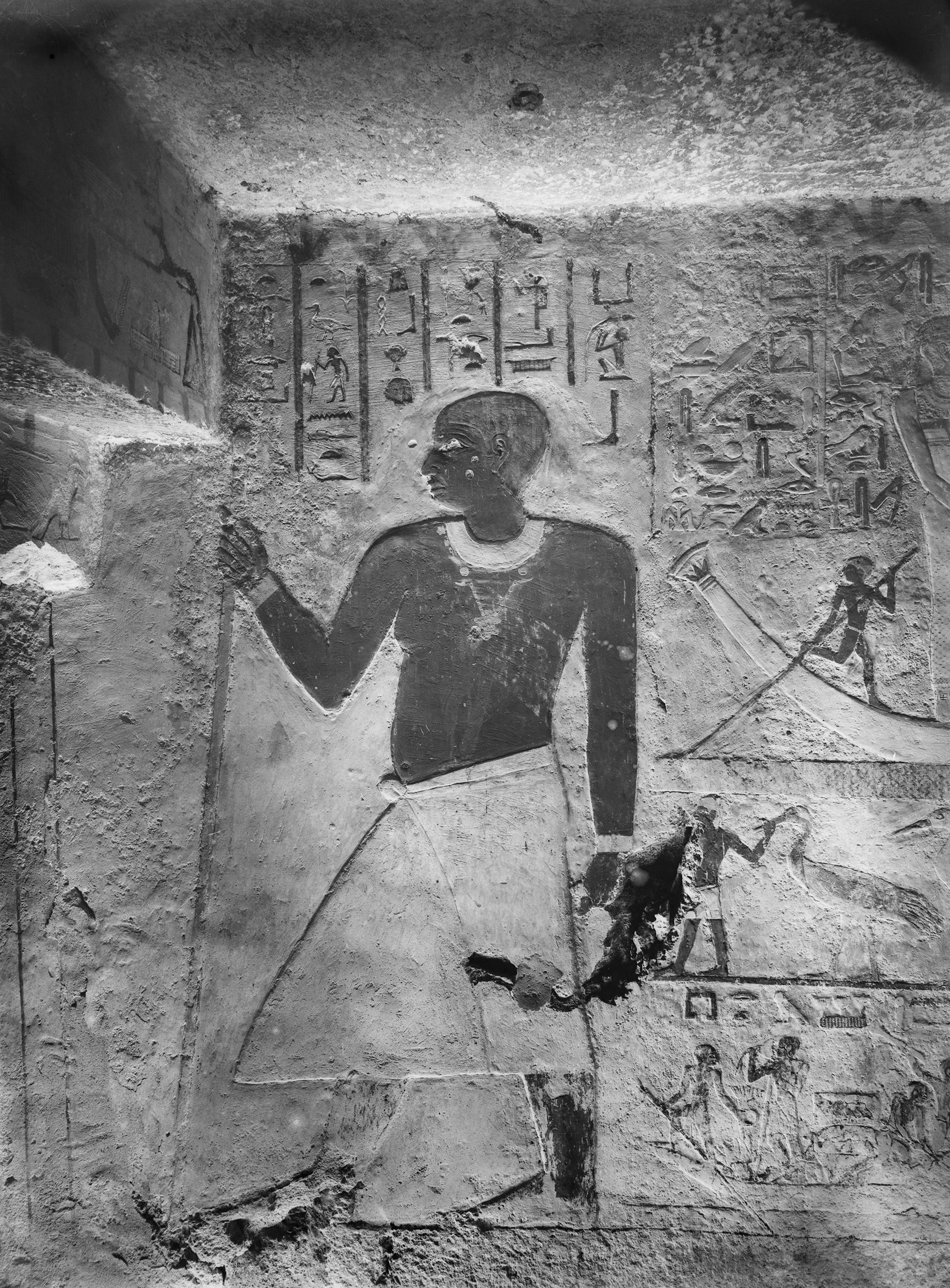This black-and-white photograph captures a detailed stone carving of an Egyptian hieroglyph, most likely found inside a cave, temple, or tomb. Central to the image is a shirtless man with a white skirt, carved in stone, who stands barefoot and looks to his left. He holds a staff in his right hand, while his left arm rests straight by his side. Surrounding him are intricate hieroglyphs, positioned at the top and to his right. The hieroglyphs above his head are small and arranged in columns, separated by lines, possibly representing different sentences or descriptions. To his right, extending from above his head to his feet, the carvings are more varied. Initially, they are chipped and faded, but below, there are smaller, detailed images: a man in a curved boat reminiscent of a gondola, using a long paddle, and another figure with what appears to be a whip or scarf in motion. Further down, an interaction between multiple figures is depicted, although eroded, making details hard to discern. Other elements include carvings of animals like birds and fish, adding to the rich tapestry of the scene. The wall itself shows signs of wear and some parts seem stained or damaged, contributing to the ancient and storied feel of the artwork.